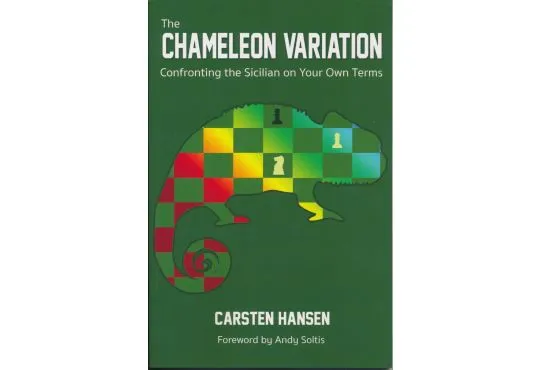The book cover for "The Chameleon Variation" by Karsten Hansen, with a foreword by Andy Soltis, showcases a striking design against a solid dark green background. Central to the cover is a silhouette of a chameleon, which contains a vibrant checkered pattern that transitions through a rainbow spectrum of colors—from dark red and purple near the tail, to orange and yellow in the middle, to light and dark green, and finally to light blue near the head. This pattern is interspersed with various chess pieces, including a white pawn in the head, a black pawn in the upper back, and a white rook near the front leg. The title "The Chameleon Variation" is prominently displayed at the top in white text, followed by the subtitle "Confronting the Sicilian on Your Own Terms." The author’s name, Karsten Hansen, along with the mention of the foreword by Andy Soltis, is also in white text at the bottom of the cover.